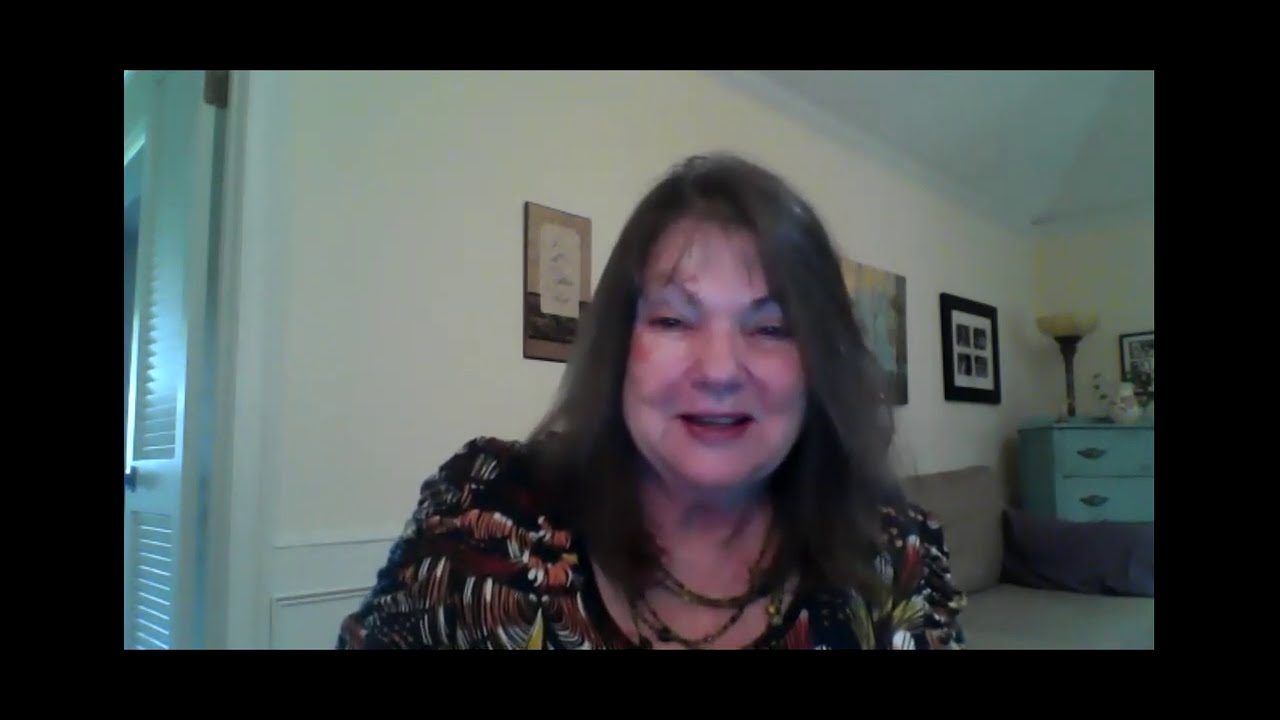The photograph is a high-definition screenshot of a video call, framed by a thick black border. At the center of the image is a woman of Caucasian descent, with shoulder-length brunette hair, slightly graying and parted to the side, featuring wispy bangs. She has almond-shaped eyes with heavy lids, very arched eyebrows, and a full bottom face accentuated by her wide cheeks. She is seen smiling, sporting berry-colored lipstick, and wearing a multicolored blouse with swirling patterns in oranges and yellows. Her outfit is complemented with several beaded necklaces. 

The background suggests a home office setting, characterized by a white wall adorned with at least three pictures and an open door with slats that allows bright sunlight to filter through. To her right, there's a blue dresser with a lamp positioned on top and other indistinct decorations. The image captures her from the chest up, giving the impression that she is engaged in a conversation through a computer camera or webcam.